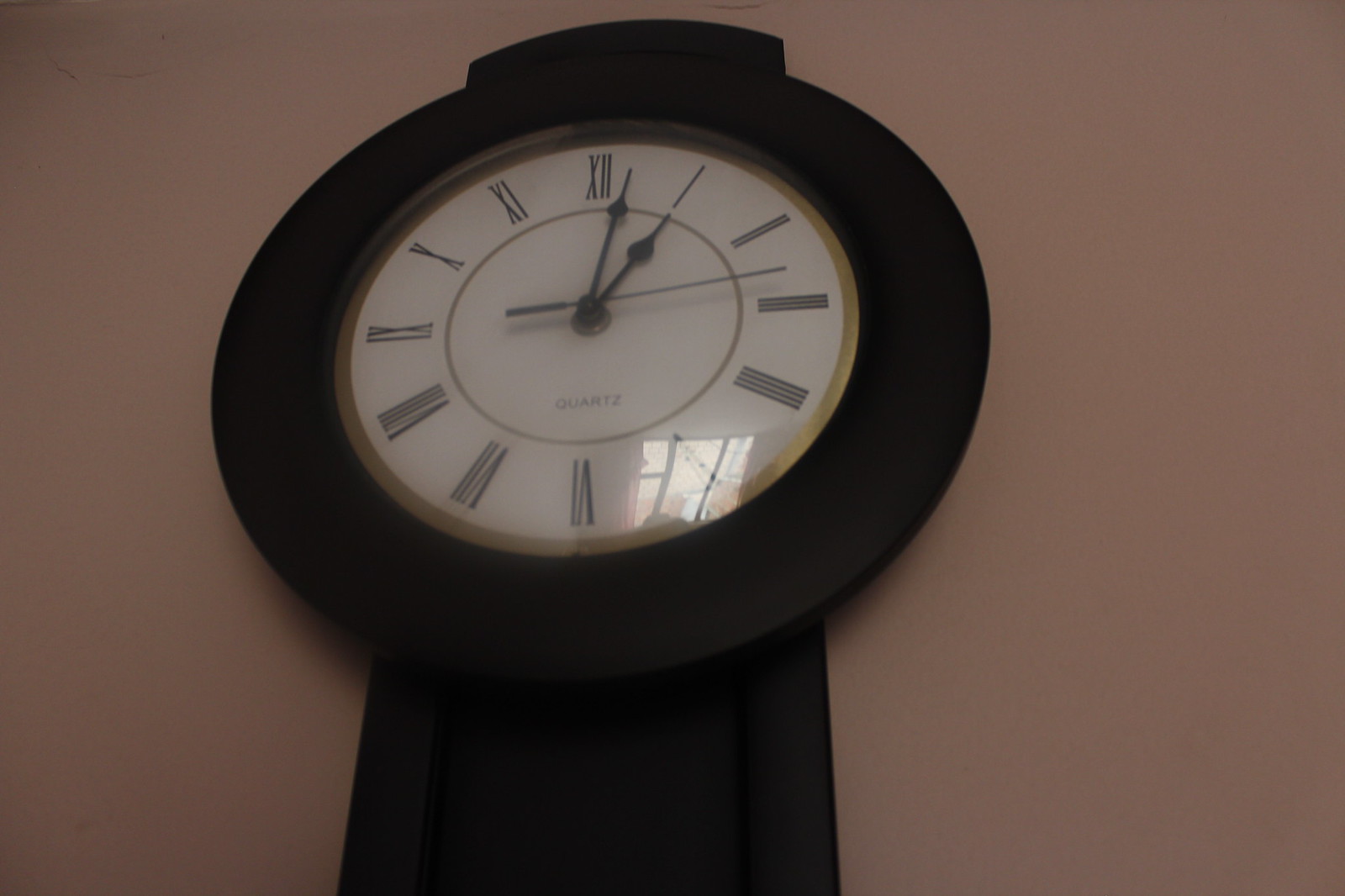In this image, we see a photograph of a wall-mounted clock, which appears to be a fusion of a grandfather clock and a more modern design. The clock is encased in a round, dark wood housing with a squared body, extending downwards, giving it a distinctive shape and presence. The wooden frame is adorned with gold trim around the outer edge of the glass-covered face, giving it a touch of elegance. The white clock face prominently displays all twelve numbers in black Roman numerals, though they may be somewhat hard to read from a distance. The clock features three black hands - the hour, minute, and second hands - with the second hand adding a dynamic touch to the otherwise steady appearance. The face also includes the word "quartz," indicating its mechanism. The background of the image shows a very light brown or dark beige wall, adding a contrasting backdrop to the dark clock. Judging from some stylistic elements, it could be inferred that this clock hails from the 1950s or 1960s. The time displayed on the clock suggests it is around 1:02 or 1:03.